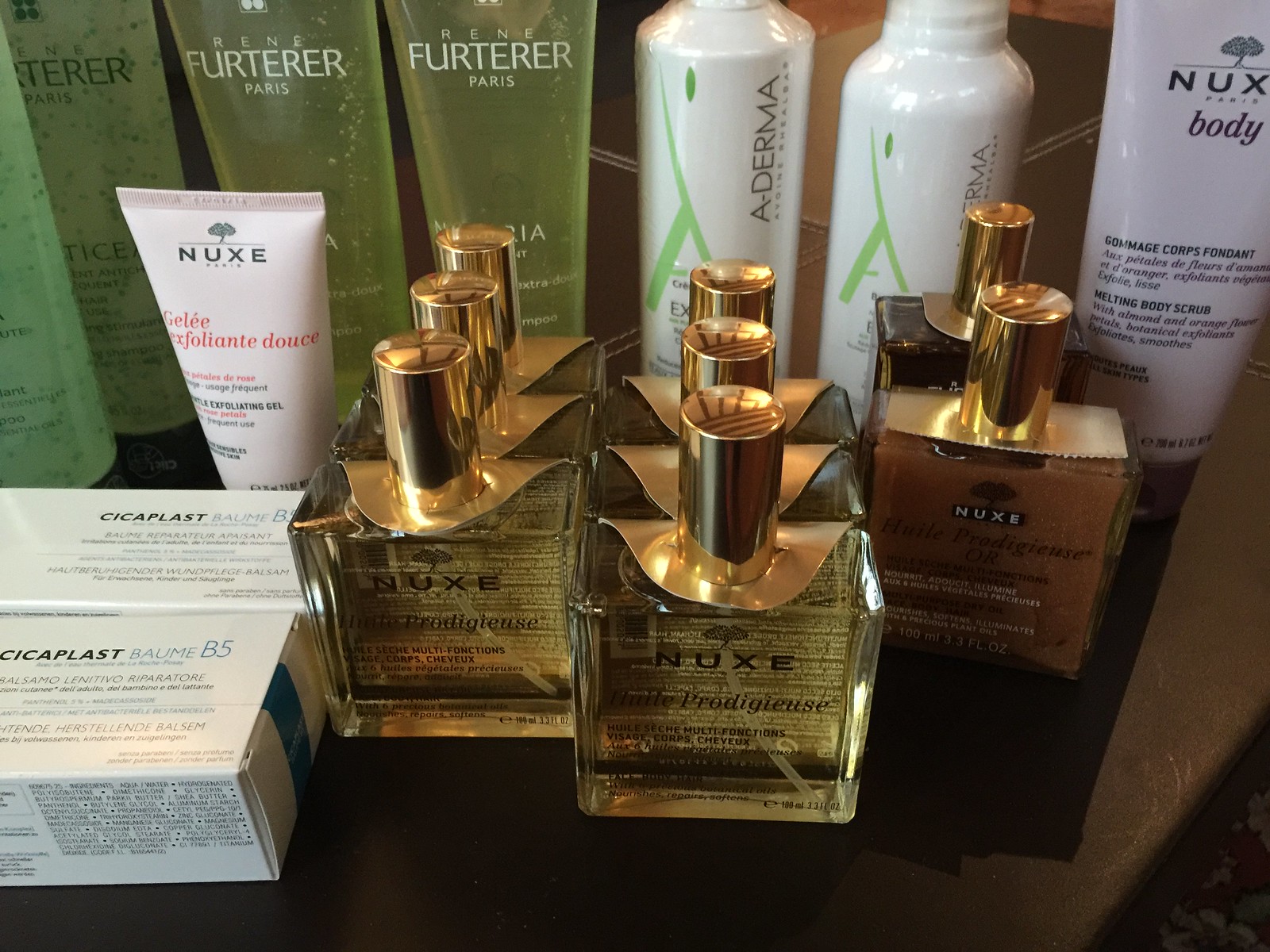The photograph showcases an orderly display of cologne bottles and skincare products on a brown shelf. Central to the image are seven square-shaped bottles of cologne from the brand NUXE, arranged in two rows of three and a single row of two. Each bottle features a clear body adorned with black lettering, including the brand name "NUXE" beneath a small tree emblem, and is topped with a gold-colored lid. The fragrance label appears to be "Elite Prodigy," written in French and accompanied by additional French text.

To the left of the cologne bottles, two unidentified flat boxes with non-English text are visible. Also present is a white tube labeled "NUXE Jelly Exfoliant" and, behind it, two translucent green tubes marked "René Furterer Paris," indicating they likely contain a gel-based product. On the right side of the shelf, there are two bottles from a brand called A-Derma, which seem to be cleansing facial scrubs. A body lotion from NUXE, also in a white tube, is positioned at the edge of the display. The overall arrangement appears neat and purposeful, suggesting a retail setting, possibly a beauty supply store or a high-end skincare boutique.